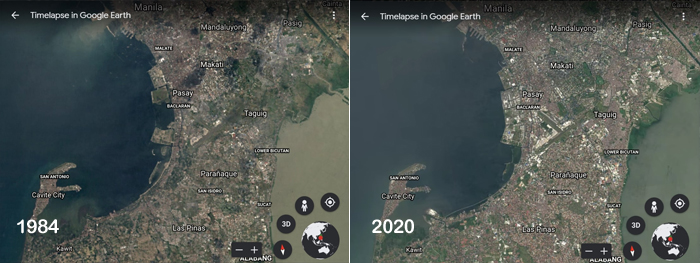The image features a time-lapse comparison from Google Earth, illustrating changes in a specific area from 1984 to 2020. Both photographs are satellite views divided into two sections: the left section dated 1984 and the right section dated 2020. The top-left corner of each image reads "time-lapse in Google Earth" in white text. The photographs depict a landscape where the right side is primarily land, showing shades of brown and green, and the left side is a bay or sea with dark blue to black water.

In the 1984 image, the landmass appears more substantial, whereas by 2020, the water has encroached, making the landmass smaller and revealing more water. This transition highlights the changes in geography over the 36-year period. Both images include white text labeling cities and towns, providing context to the mapped area. At the bottom right of each photograph are four black circular buttons part of the Google Earth interface, alongside a partial image of a white and black Earth icon, suggesting different view options within the software. Notable differences between the images include more prominent white areas in the 2020 map, indicating potential developments or changes in terrain.